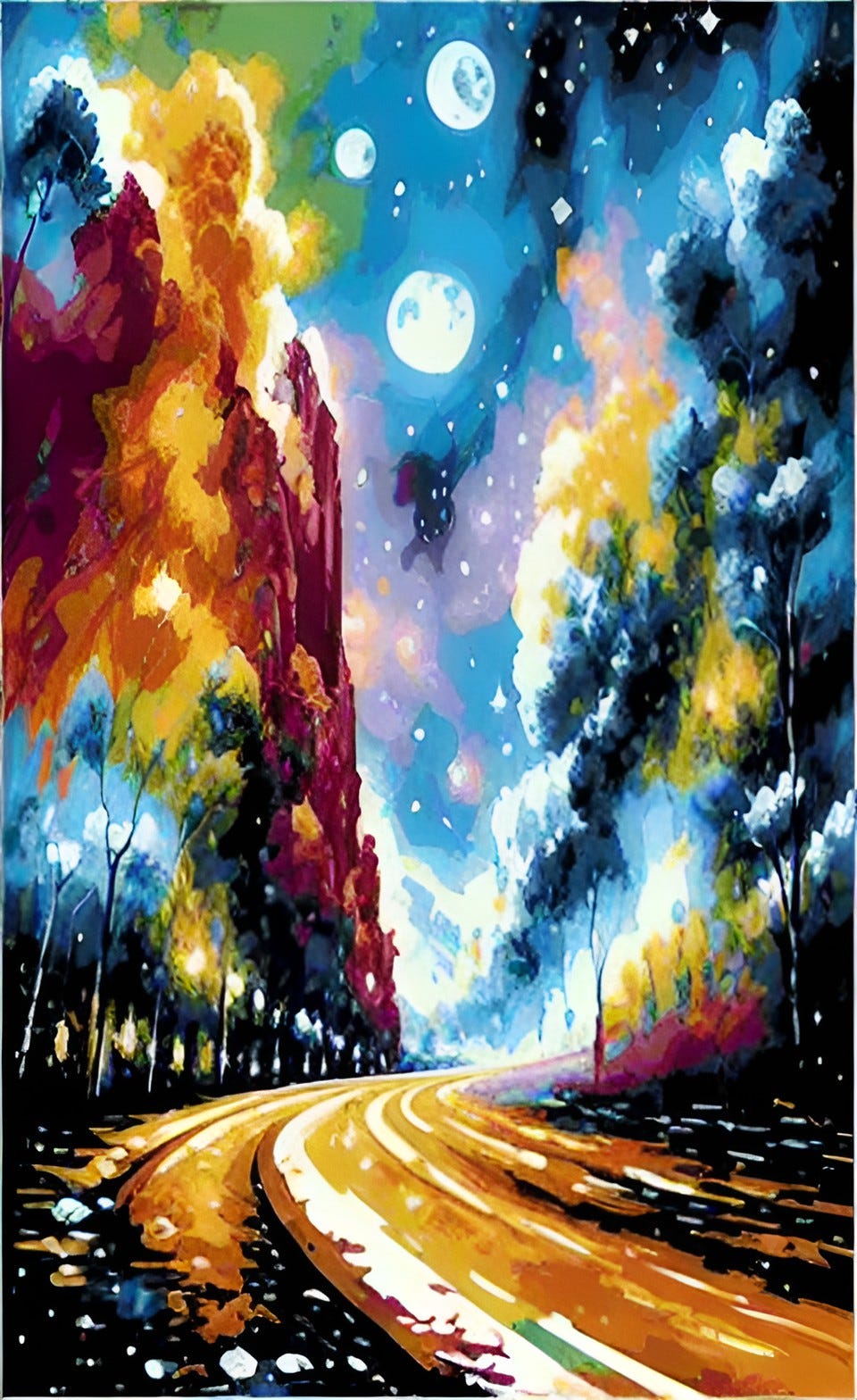This image is a slightly abstract, psychedelic night scene, rich in vibrant, diverse colors. The street, depicted in a blend of orange, white, and black, is lined with trees on both sides. The trees exhibit a kaleidoscope of hues including light and dark reds, burnt oranges, blacks, light greens, lavenders, blues, yellows, and dark blues, creating a striking visual contrast. On the left side of the image stands a solitary street lamp, adding to the night's ambiance. The sky is dark, interspersed with greens and adorned with three celestial circles—one large, one medium, and one smaller—symbolizing stars or moons. These circles, arranged with the smaller one positioned slightly to the left, illuminate the scene with a cosmic glow. The entire artwork, possibly done with acrylic paint, conveys a surreal and beautifully blended pathway that invites viewers into a dreamlike, universal exploration.